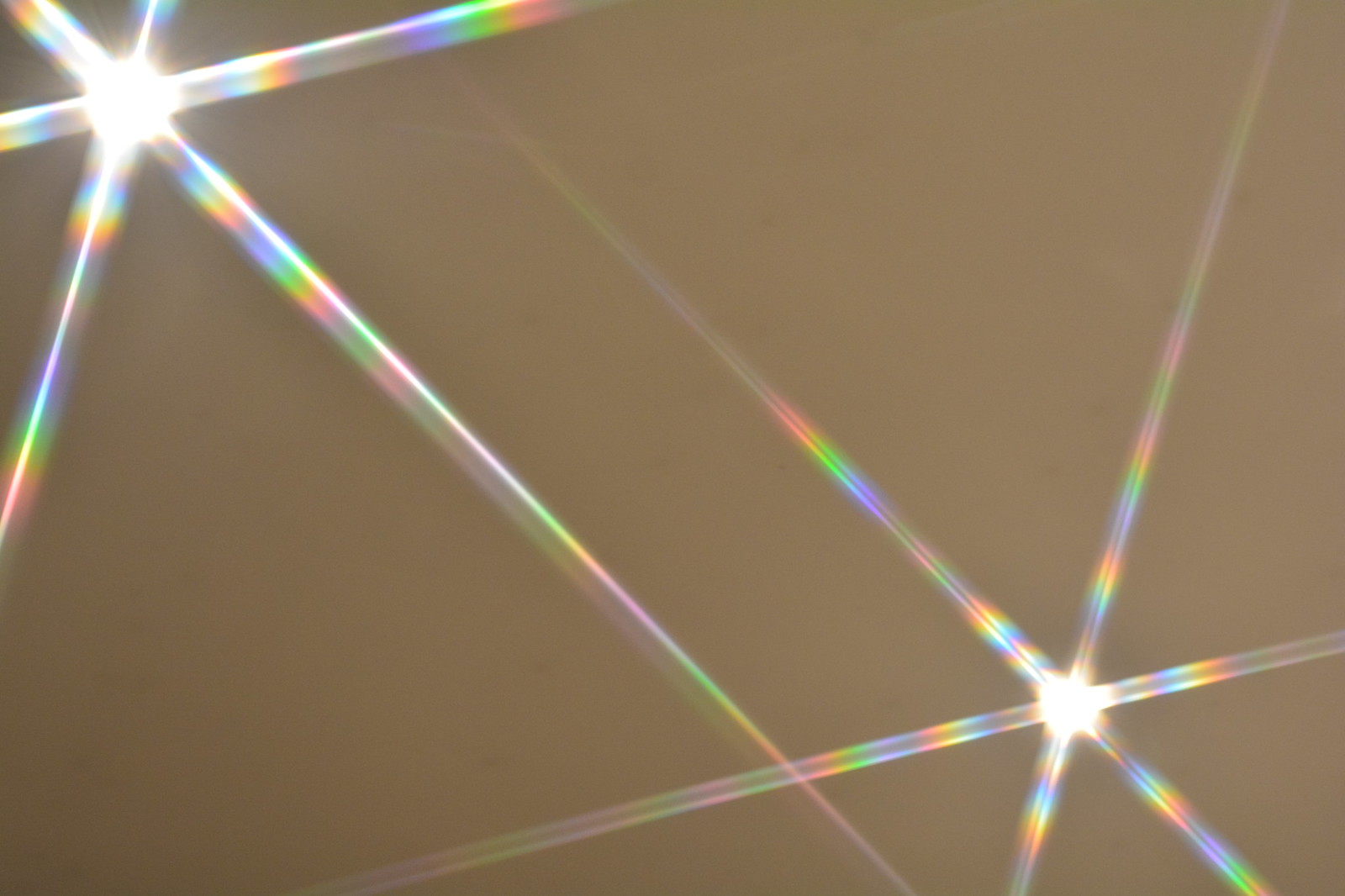This color photograph, taken indoors against a beige-brown backdrop, likely intended as an artistic piece, features two ceiling lights positioned in the upper left and lower right corners. The lights create intricate star-shaped patterns, each emitting six prism-like beams in vibrant colors spanning the visible light spectrum—red, yellow, green, blue, and purple. These prismatic beams intersect at the center, surrounded by a brilliant white light. The straws of light, as they stretch diagonally across the image, almost meet but do not fully connect from corner to corner, forming X-like shapes in the visual composition. The picture is captured from floor level, offering a unique perspective on the ceiling setup.